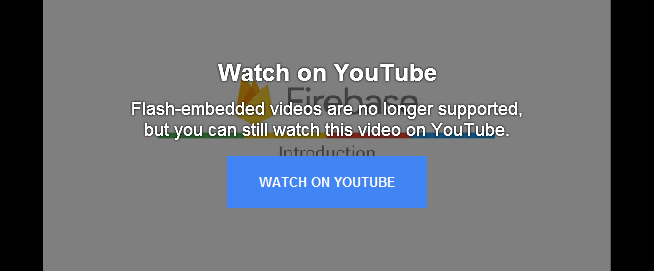The image is a screenshot of a webpage overlaid with a semi-transparent gray shade. In the center of the gray overlay, white text reads: "Watch on YouTube. Flash embedded videos are no longer supported, but you can still watch this video on YouTube." Below this text is a prominent blue button labeled "Watch on YouTube," inviting users to click and view the video on the YouTube platform.

In the background, partially obscured by the gray overlay, is the Firebase logo. This logo features a stylized flame next to the word "Firebase." Directly underneath the logo is a series of colorful horizontal bars. From left to right, the colors of these bars are green, yellow, orange (resembling a flame), red, and blue. Beneath these colorful bars is the word "Introduction," indicating the section or content being described.

The borders on either side of the main content area are solid black, framing the entire image.